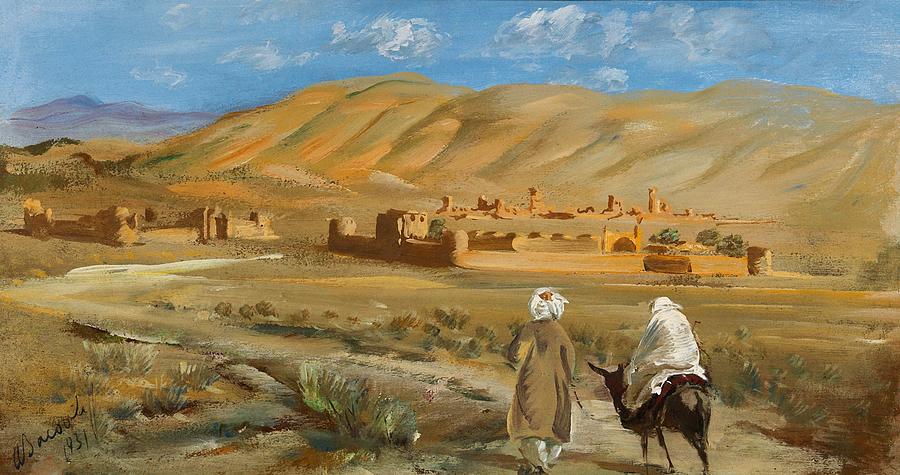The painting depicts a vast desert landscape under a clear blue sky dotted with wispy grayish-white clouds. In the foreground, a man in a white and gold tunic, with flowing harem-style balloon pants and a white turban, leads a donkey carrying a cloaked figure dressed entirely in white. The pair tread along a winding, sandy path surrounded by patches of dried grass and low-growing shrubs. The path meanders toward a distant, low and flat city, seemingly constructed from sandstone, giving it a natural, earthy appearance. Behind the city, a series of yellow and tan hills stretches across the horizon, with a purplish mountain emerging in the far left distance. In the center of the scene are structures resembling ruins or low buildings, surrounded by walled compounds and sparse shrubbery. The painting, likely an oil painting on canvas or board, evokes a sense of ancient times, possibly as a biblical illustration, emphasizing the timeless and historical atmosphere of the depicted landscape.